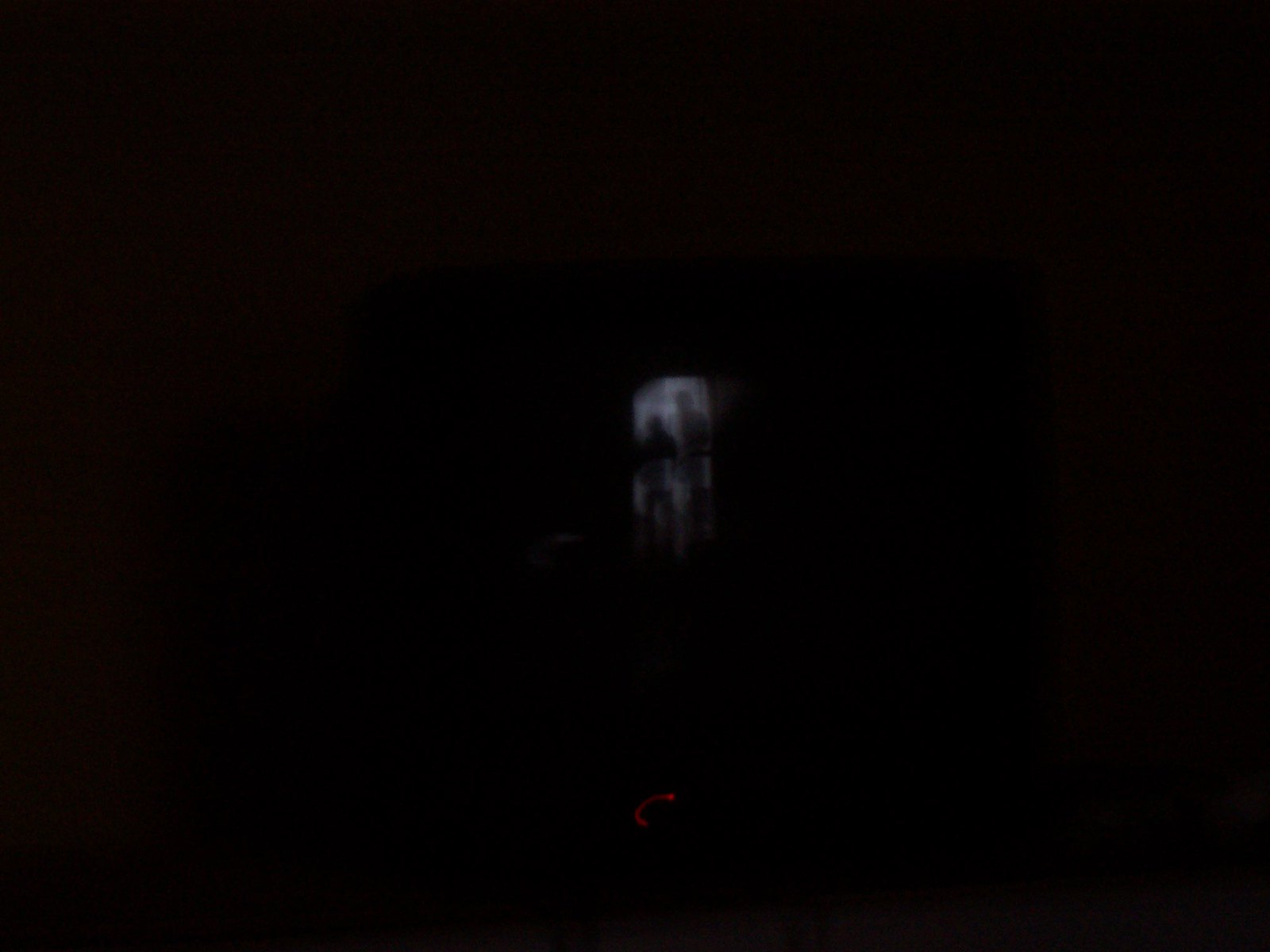The image is extremely dark and mostly black with very little detail visible. At the center of the image, the only source of light reveals what appears to be two people, or perhaps a person and their shadow, standing next to each other. The forms are small, blurry, and gray-blue in color against the dark backdrop, making it difficult to distinguish specific features or actions. Below this central light, near the bottom of the image, there is a small, dimly lit red semicircle. The overall impression is one of indistinct silhouettes amidst a nearly opaque background, with minimal additional detail discernible.